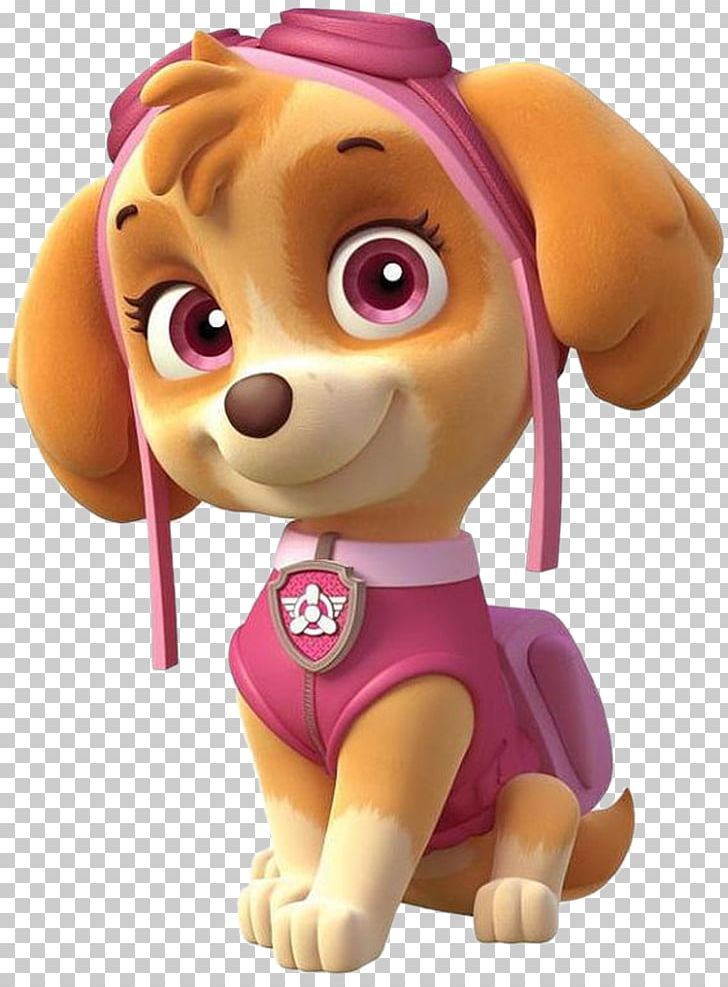This image is a highly detailed 3D render of Skye, a character from Paw Patrol. Skye is depicted in a cartoony style and resembles a brown Cocker Spaniel. Her fur is primarily brown, with lighter, pale yellow or light beige patches on her paws and around her mouth. Skye has large violet eyes accented with black eyelashes and black eyebrows that hover above them. She sports fluffy brown ears and a tuft of hair on her head. 

Skye is outfitted in pink goggles perched on top of her head, a pink vest, and a pink backpack. There is a collar around her neck featuring a symbol that resembles a Mercedes-Benz logo. She is smiling and looking directly at the camera. The background of the image is a transparency style with a white and brown checker pattern. Overall, the image is a stylized, artist's rendition that could be mistaken for a toy or an anime character, designed to appeal to children.